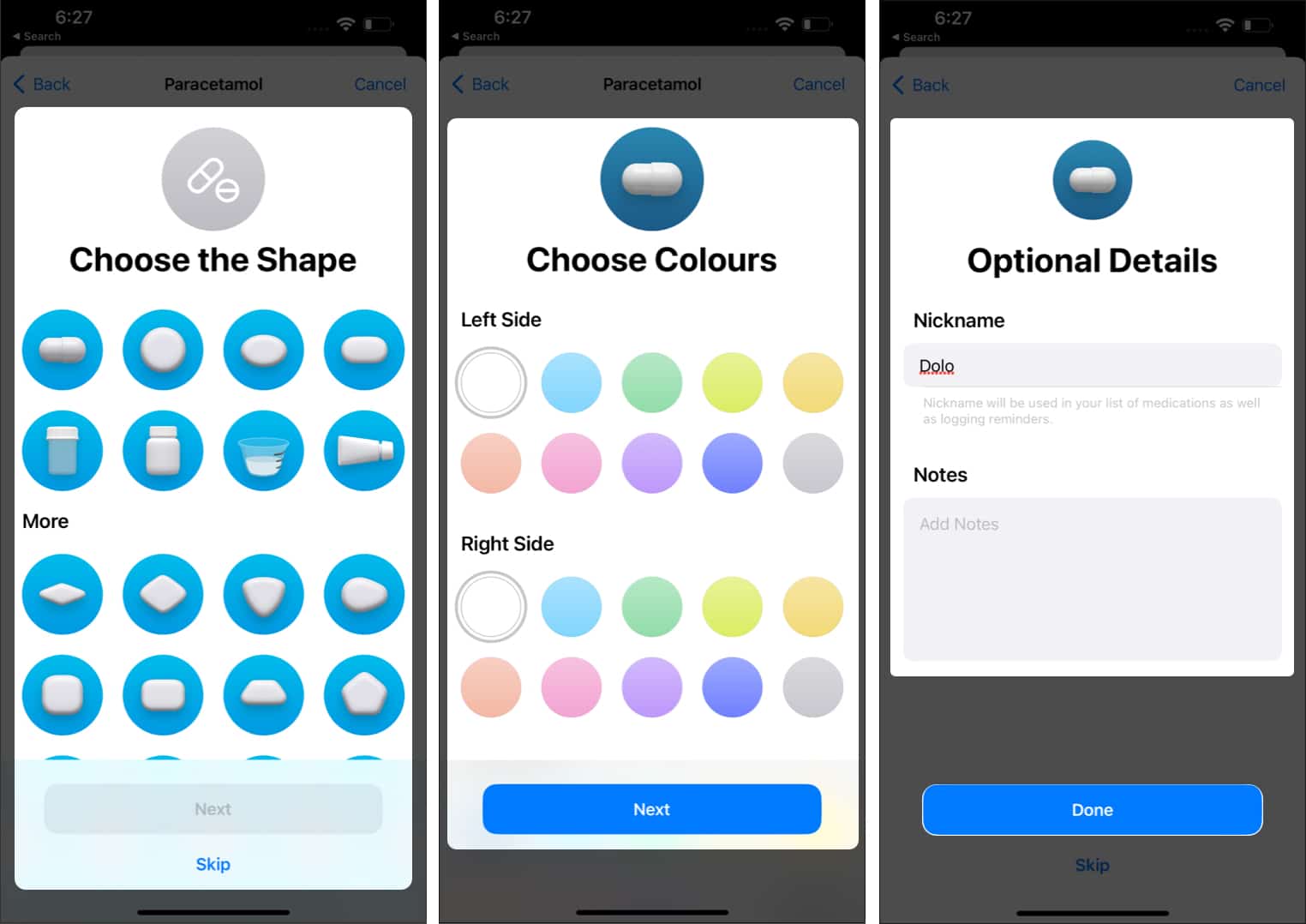The image depicts a screen with a grey header, showcasing two types of pills: one oval and one round. The header text reads "Choose the shape." Below it, in blue text, various shapes are listed, including capsule, round, oval, oblong, bottle with a white cap, white medicine bottle, a measuring cup like those used for cough syrup, a cheerleader megaphone, a diamond, a larger diamond, a triangle, a square, and a rectangle.

The background of the screen is grey, with "Next" and "Skip" options in blue font. 

The screen then prompts the user to "Choose colors," dividing the interface into two sections: left and right. On the left side, available colors are white, blue, green, yellow, a brighter yellow, orange, pink, purple, blue, and grey. On the right side, the colors listed are white, blue, green, yellow, orange, another shade of orange, pink, purple, blue, and grey. "Next" follows after these options.

Further down, the screen has a section for "Optional details." There is a field labeled "Nickname," with the example "dolo" underlined in red, indicating that the nickname will be used in the user's list of medications and for logging reminders. Another field, labeled "Notes," appears in grey with the placeholder text "add notes."

At the bottom of the screen, the options "Done" and "Skip" are presented in blue text.